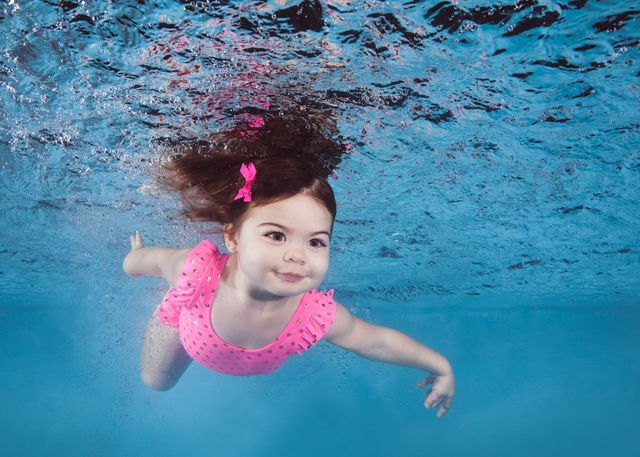This photograph captures a heartwarming moment underwater in a swimming pool, featuring a small girl who appears to be about two years old. She has a pile of brown hair, partially tied back with a pink bow, and her hair is fanning out in the water. Her large, wide-open eyes and slightly smiling expression, with her lips firmly closed, reflect both a sense of curiosity and delight. The little girl is adorned in a pink one-piece bathing suit with silver polka dots, contrasting beautifully against the surrounding blue water. Her orientation in the rectangular image shows her more on the left side, with her left arm extended forward, indicating she is actively swimming, while her right arm trails behind her. The surface of the water above her is a vibrant blue, marked with ripples and reflections that add to the dynamic feeling of the scene. The image captures her just below this reflective surface, showcasing her big eyes and cheeks, and the overall effect is one of pure, captivating innocence.